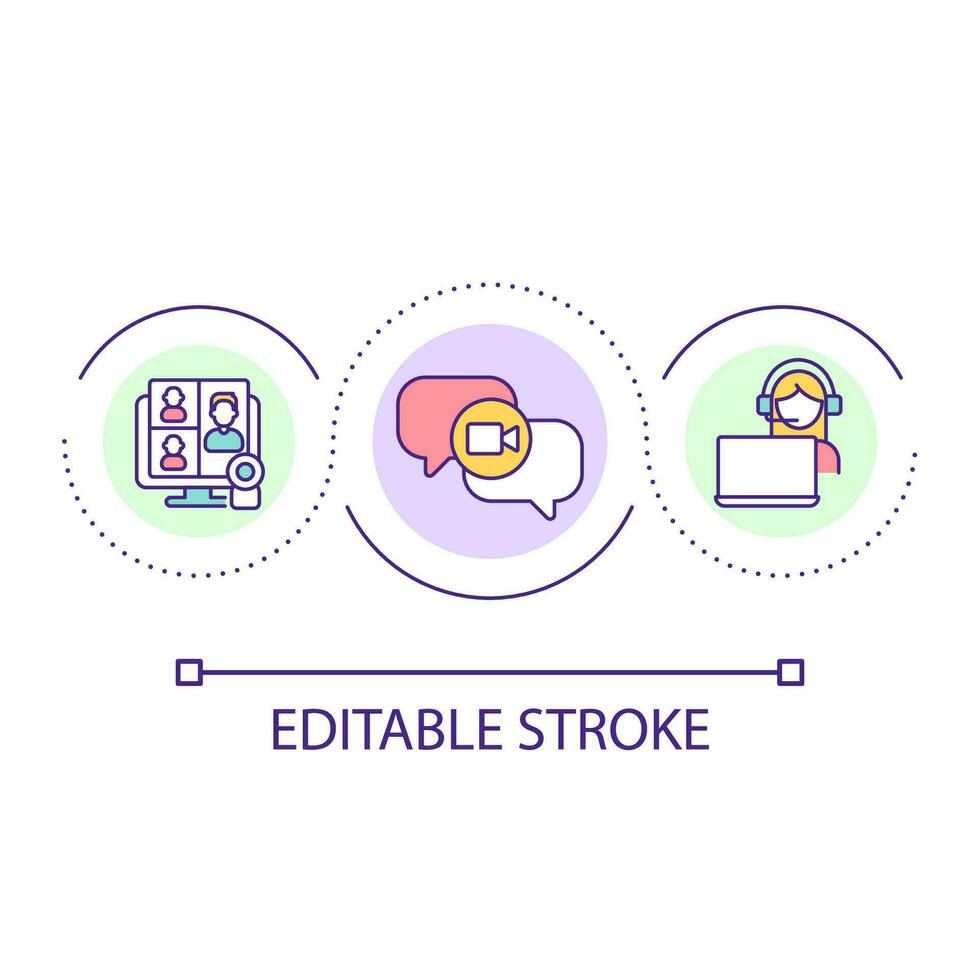In this image, we see an animated-style diagram set against a white background, prominently featuring the phrase "editable stroke" in large purple text at the bottom. Above this text, a solid purple line stretches horizontally, terminating in small purple squares at each end. Positioned above the line are three interconnected circular illustrations. The leftmost circle displays a computer monitor showing three figures: one adult (in blue) and two children (in pink). The middle circle depicts two overlapping text message icons with a small video chat camera icon, suggesting communication or a FaceTime interaction. The rightmost circle, set against a green background, features a woman with long blonde hair and headphones, working on a laptop. The overall diagram incorporates a blend of purple, lilac, green, pink, and gold tones.